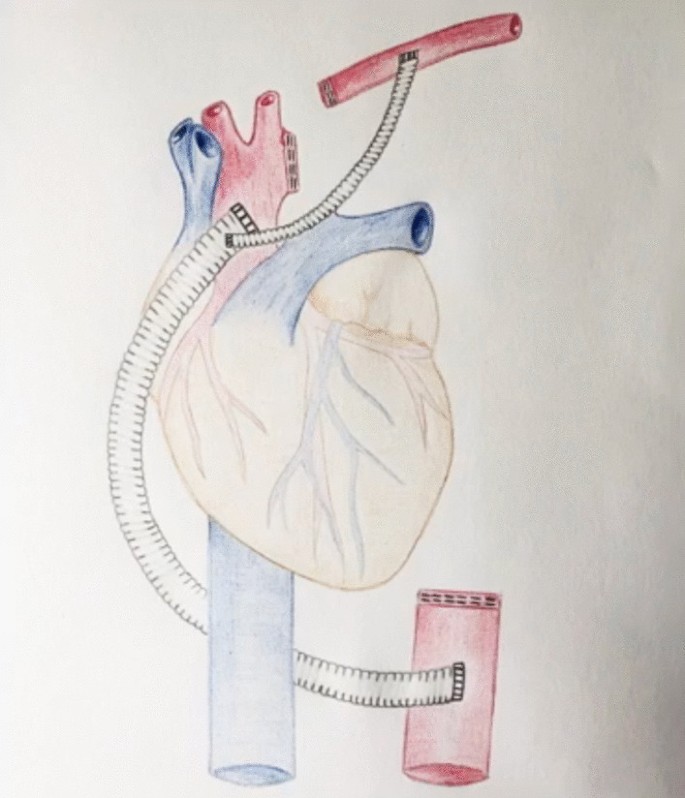This is a detailed and colored pencil illustration of an anatomically correct human heart. The heart is primarily depicted in a light, pale brown, almost white hue, and is positioned slightly to the left center of the image. Prominently featured are three large valves: two blue valves and one red valve, along with blue veins and red arteries. The tubes and pipes attached to the heart give the appearance of an early invention or artificial modification. One blue valve leads to an unusually straight blue tube, and another tube seems to wrap around the heart, connecting differently colored sections. This tube is reminiscent of a handle. The configuration includes a red valve connected to a man-made looking red tube section, illustrating artificial interventions possibly in the early stages of design. The heart is surrounded by these tubes, with three valves positioned at the top and another at the bottom, all intertwined around the heart, particularly near the upper and center regions.